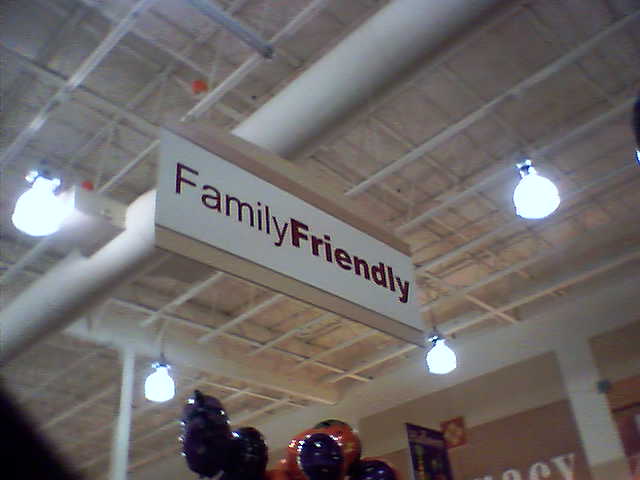Inside a store, the photograph captures a view looking up at the ceiling, revealing an intricate network of metal rafters and various pipes, prominently featuring large white pipes. Suspended from the ceiling are several large, white lights, illuminating the space below. A beige sign with brown writing reads "FAMILY," and in thicker brown letters, the word "FRIENDLY" stands out beneath it. In the background, there is a dark brown wall, partially obscured by the angle of the shot, with only the tips of some letters visible, making them unreadable. Additionally, a blue sign hangs nearby, and in the middle of the space, a cluster of round, shiny balloons can be seen. The balloon arrangement includes three blue balloons, accompanied by several large orange and blue balloons.